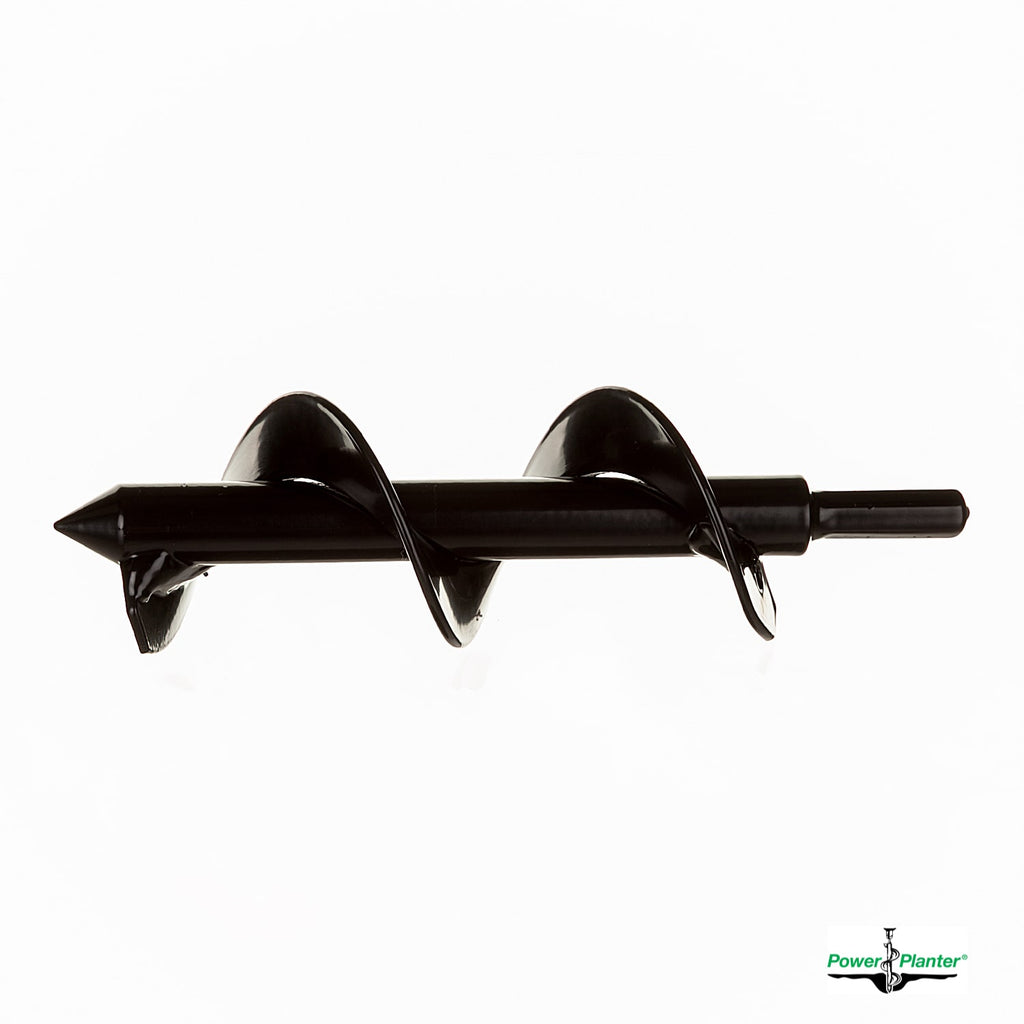The image displays a black auger drill bit prominently set against a plain white background. The bit itself, constructed from shiny black steel, features a pointed end akin to a pencil. The long rod is wrapped with a spiral, flat metal designed to dig into the soil, resembling DNA strands in its helical structure. The opposite end of the bit has a hexagonal shape, which would fit into a power drill or battery-powered device, making it ideal for digging holes for planting, tilling, or uprooting. In the bottom right corner of the image, the Power Planter logo is visible, depicted in green font alongside a black emblem of an auger bit standing upright. This visual composition suggests that the image is likely used for advertising the Power Planter tool.